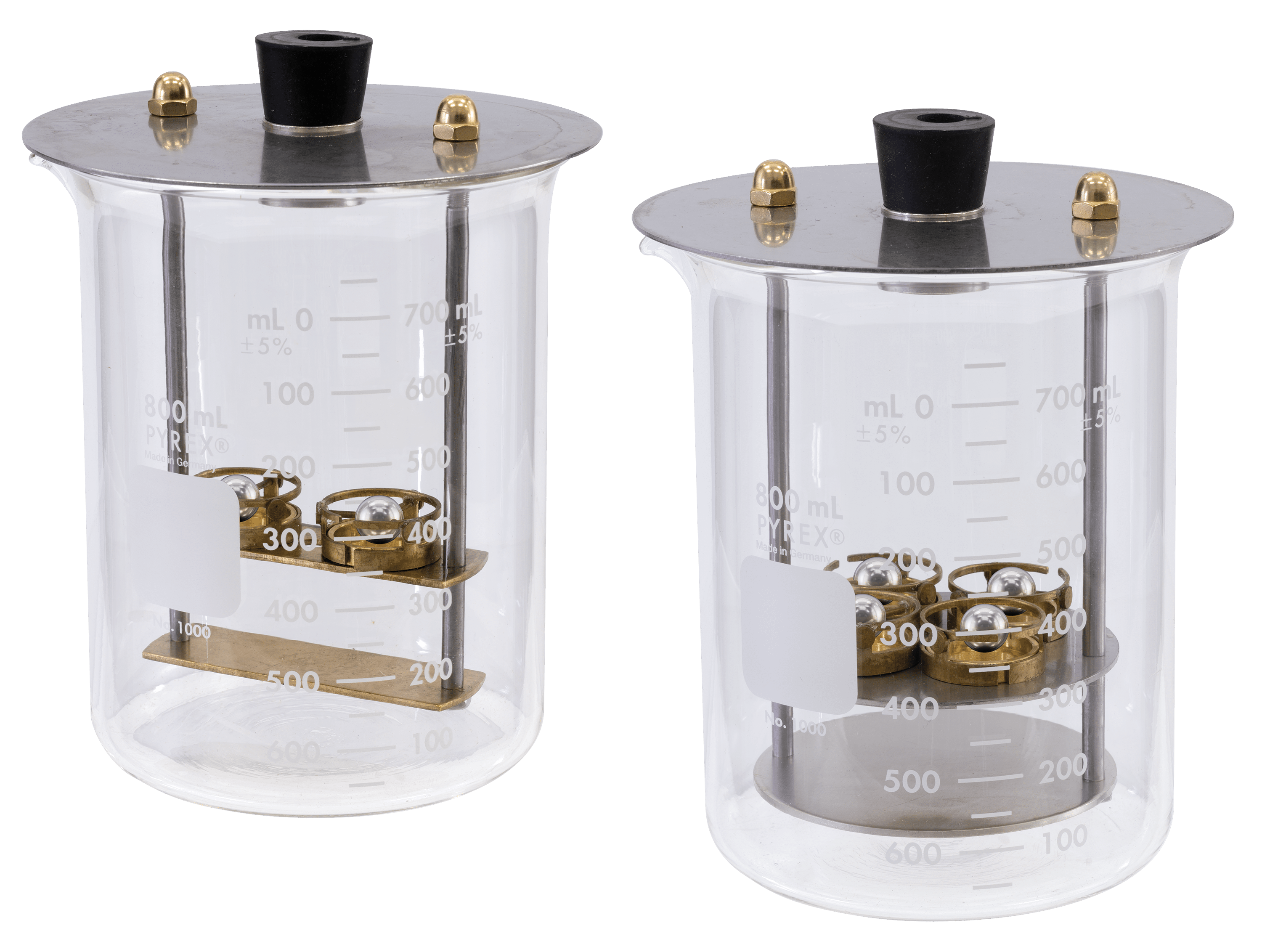A detailed product photograph showcases two pieces of scientific equipment, prominently featuring glass beakers standing on a white background, possibly intended for retail purposes on a website. Each glass beaker is labeled with milliliter measurements, ranging from 0 to 700 milliliters, in increments of 100 milliliters. The beakers have metal lids attached to them, secured with two gold-colored bolts or brass inserts. These lids are composed of steel and have threaded rods extending from them into the interior of the beakers.

Inside each beaker are metallic structures designed to hold various contents. The beaker on the left features a configuration that resembles thin, rectangular shelves or a swing set, hosting two copper-colored disks, each containing a steel-colored ball bearing. In contrast, the right-hand beaker includes four circular, metal shelves, each also containing a copper-colored disk with a steel ball bearing.

These detailed apparatuses suggest that the equipment is used for scientific experiments or precise measurements involving liquids and possibly other materials, highlighting their potential use in laboratory settings.